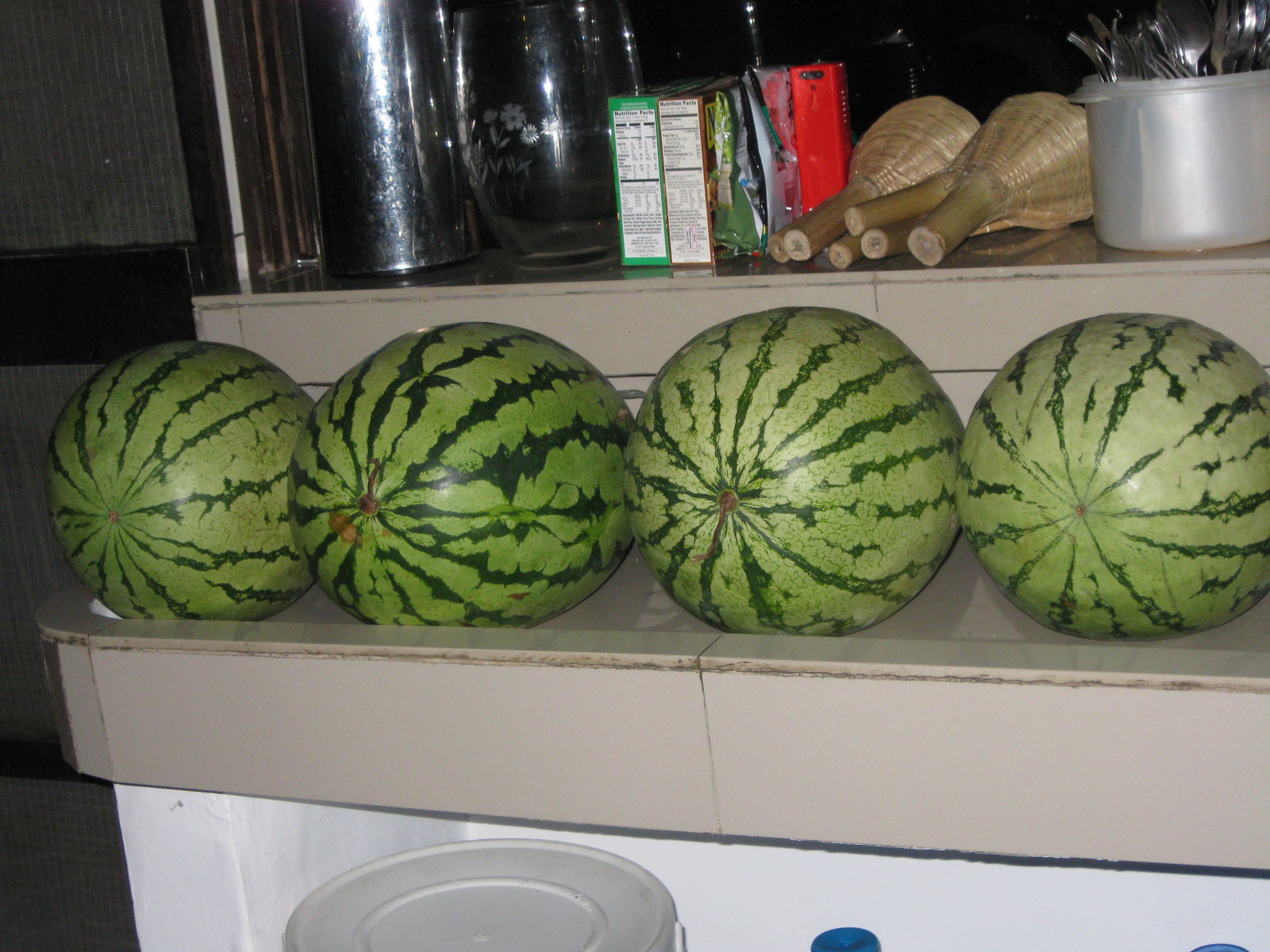This image features a front-on view of a countertop with two tan and white shelves. On the light pink countertop, which appears cluttered and somewhat dirty, sit four large, whole cannonball watermelons. These watermelons display two-tone green stripes, with the one second from the left having darker stripes indicating potential unripeness. The melons are arranged horizontally, with the stem ends of the two central melons visible. Below the counter, a lidded five-gallon bucket is partially visible. The upper shelf holds a variety of items, including small boxes of food, possibly rice, a couple of conical baskets, a silver container filled with utensils, a chrome cylindrical container, a round holder with utensils, and a glass vase. The scene is detailed with various elements, contributing to an overall sense of organized yet cluttered storage.